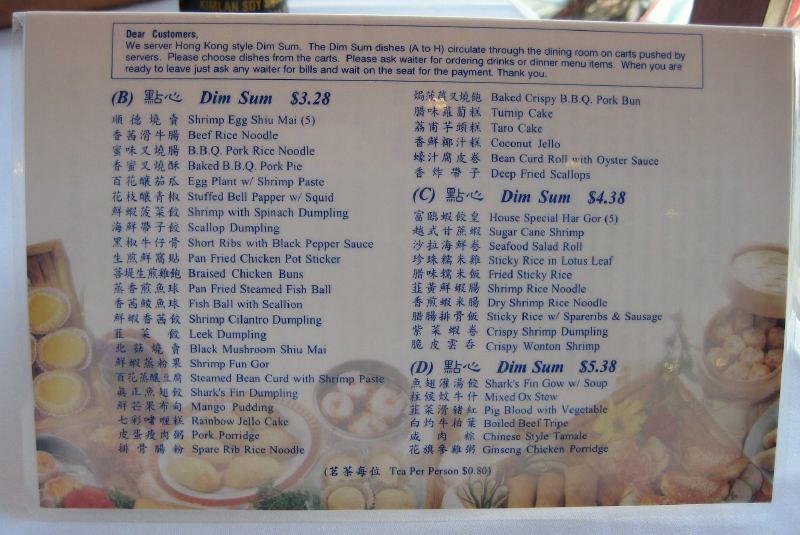The image showcases a detailed dim sum menu at a restaurant specializing in Hong Kong-style dim sum. At the top, the menu warmly addresses customers: 

"Dear Customers, we serve Hong Kong-style dim sum. The dim sum dishes, labeled from A to H, circulate through the dining room on carts pushed by servers. Please choose dishes from the carts. If you wish to order drinks or items from the dinner menu, ask any waiter. When you are ready to leave, ask any waiter for the bill and remain seated for payment. Thank you."

Following this introduction, the menu lists a variety of dim sum offerings categorized by price points:

**$3.28 Dim Sum:**
- Shrimp Egg Shumai
- Beef Rice Noodle
- Barbecue Pork Rice Noodle
- Baked Barbecue Pork Pie
- Eggplant with Shrimp Paste
- Stuffed Bell Pepper with Squid
- Shrimp with Spinach Dumpling
- Scallop Dumpling
- Short Ribs with Black Pepper Sauce
- Pan-Fried Chicken Pot Sticker
- Braised Chicken Buns
- Pan-Fried Steamed Fish Ball
- Fish Ball with Scallion
- Shrimp Cilantro Dumpling
- Leek Dumpling
- Black Mushroom Shumai
- Shrimp Fungor
- Steamed Bean Curd with Shrimp Paste
- Shark's Fin Dumpling
- Mango Pudding
- Rainbow Jello Cake
- Pork Porridge
- Spare Rib Rice Noodle
- Baked Crispy Barbecue Pork Bun
- Turnip Cake
- Taro Cake
- Coconut Jello
- Bean Curd Roll with Oyster Sauce
- Deep-Fried Scallops

**$4.38 Dim Sum:**
- House Special Har Gow
- Sugar Cane Shrimp
- Seafood Salad Roll
- Sticky Rice in Lotus Leaf
- Fried Sticky Rice
- Shrimp Rice Noodle
- Dry Shrimp Rice Noodle
- Sticky Rice with Spare Ribs and Sausage
- Crispy Shrimp Dumpling
- Crispy Wonton Shrimp

**$5.38 Dim Sum:**
- Shark’s Fin Go with Soup
- Mixed Ox Stew
- Pig Blood with Vegetable
- Boiled Beef Tripe
- Chinese Style Tamale
- Ginseng Chicken Porridge

This comprehensive menu offers an array of traditional and specialty dim sum dishes, catering to diverse palates and preferences in the dining room setting.